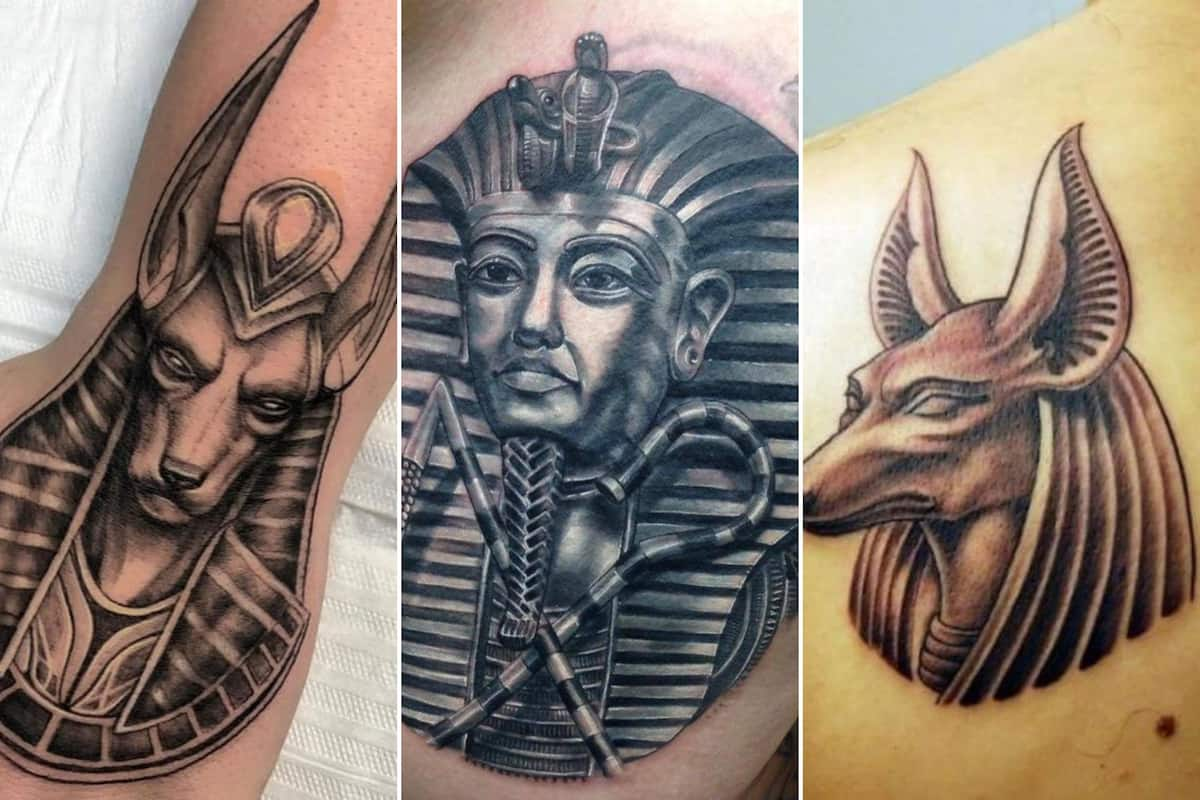The image consists of three separate panels of equal dimensions, each featuring a detailed photograph of a tattoo on human skin, all centered around ancient Egyptian themes. 

In the leftmost panel, against a white cloth background, is a tattoo on the back of a person's hand, depicting the face of Anubis, the Egyptian god with long ears, situated on a shield. This tattoo is on a lightly tanned Caucasian arm.

The middle panel shows a tattoo of an Egyptian pharaoh with a coffin headdress. The intricate tattoo predominantly uses black and silver hues and appears to be on a paler part of the body, possibly a knee or an arm, though its exact location is unclear.

The rightmost panel features another Anubis tattoo, this time in a three-quarter profile with slightly shorter ears than the first. This tattoo is rendered in a brown color on a more yellowed skin tone.

The tattoos, each with serious facial expressions, emphasize the gravity and reverence associated with their ancient Egyptian subjects.